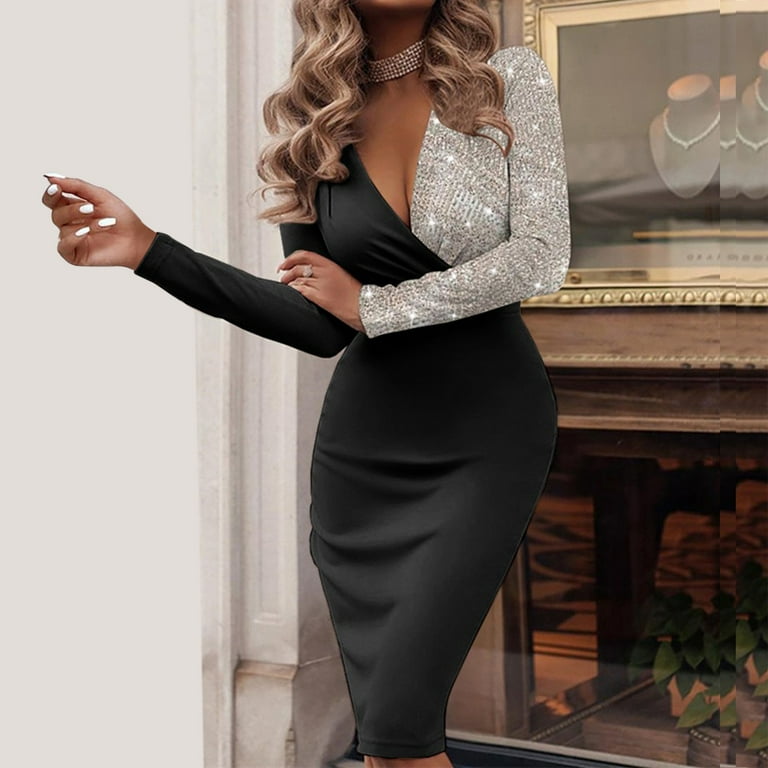This photograph portrays a stylish, dark-skinned woman standing in a white room, likely next to a fireplace. She is dressed in a form-fitting, knee-length black dress with a striking contrast: the right side is entirely black, while the left arm and shoulder are adorned with glittering silver sequins. Her attire includes a layered, ornate choker necklace sparkling with rhinestones. She has long, wavy blonde hair cascading down, and her nails are painted a bright white. The background features a large, gold-framed painting or photograph, reflecting several mannequin necks displaying necklaces.